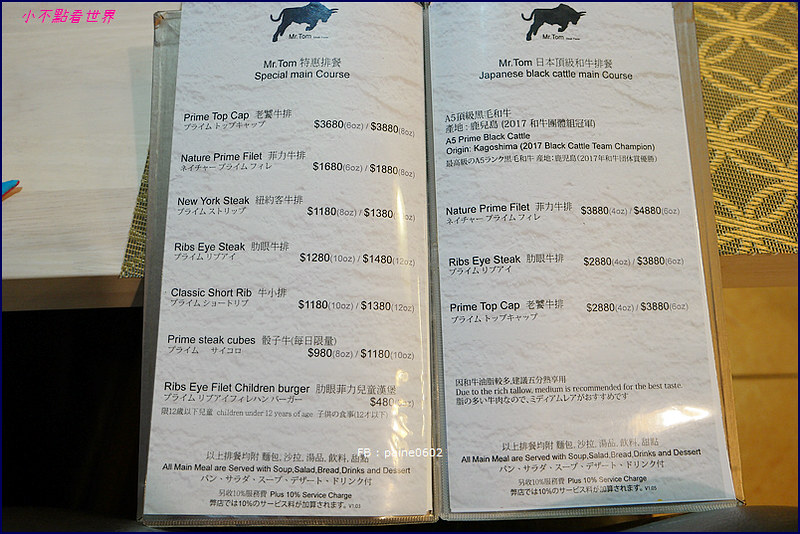The image features a meticulously arranged two-page menu from a steakhouse named "Mr. Tom's." Each page prominently displays a striking black illustration of a charging bull at the top, signifying the restaurant's robust and hearty fare. The menu pages are encased in a glossy page protector, adding a subtle sheen to the content. The background of the pages mimics a refined marble design, lending an air of sophistication to the presentation.

On the left page, "Mr. Tom's Special Main Course" section lists seven delectable items, starting with the "Prime Top Cap," each accompanied by distinct prices. The right page showcases the "Prime Black Cattle" selection, also with varying prices for each dish. Various accompaniments that come with the meals are briefly described at the bottom.

Near the top right corner of the left page, a touch of Asian influence is evident with some writings in pink, while additional Asian characters are scattered throughout the menu. The setting of the image includes a glimpse of a rich, brown table adorned with a green and gold-patterned tablecloth, enhancing the elegant aesthetic of the scene. The attention to detail in the menu design and the subtle multicultural elements suggest a dining experience that is both luxurious and globally inspired.